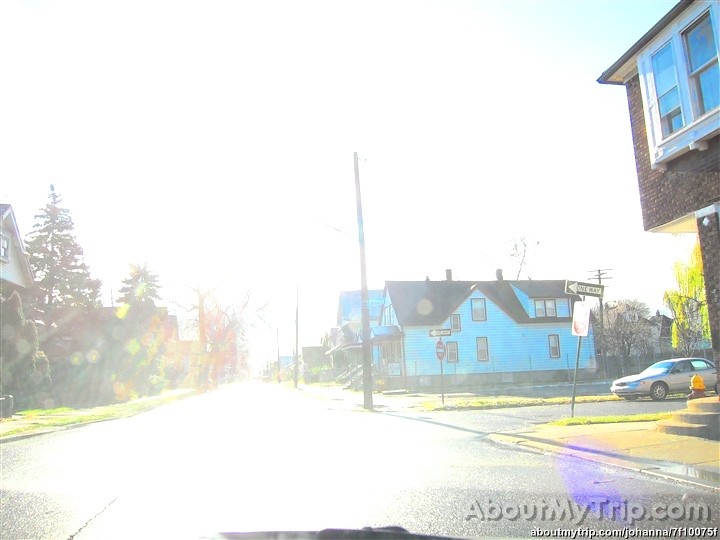This daytime photograph captures a tranquil residential neighborhood with a variety of features that add depth and character to the scene. A noticeable lens flare effect gives the image a slightly dreamy quality. At the bottom, a watermark reads "aboutmytrip.com/j-o-h-a-n-n-a" followed by a string of letters and numbers.

In the foreground, the pavement of the street is clearly visible, bordered by well-maintained green grass. Street signs are present, including one-way signs with a black background and white arrows directing traffic. A silver car is parked along the street, adding a touch of everyday life to the scene.

A gray and yellow fire hydrant stands out, offering a splash of color amidst the greenery. Two houses dominate the background: one is a quaint brick house, and the other is a large white house with a contrasting dark-colored roof. 

Nature graces the neighborhood with an array of trees, some full with green leaves and others bare, hinting at seasonal change. Power poles line the street, adding to the suburb’s infrastructure. The overall composition presents a peaceful slice of suburban life, rich with detail and variety.